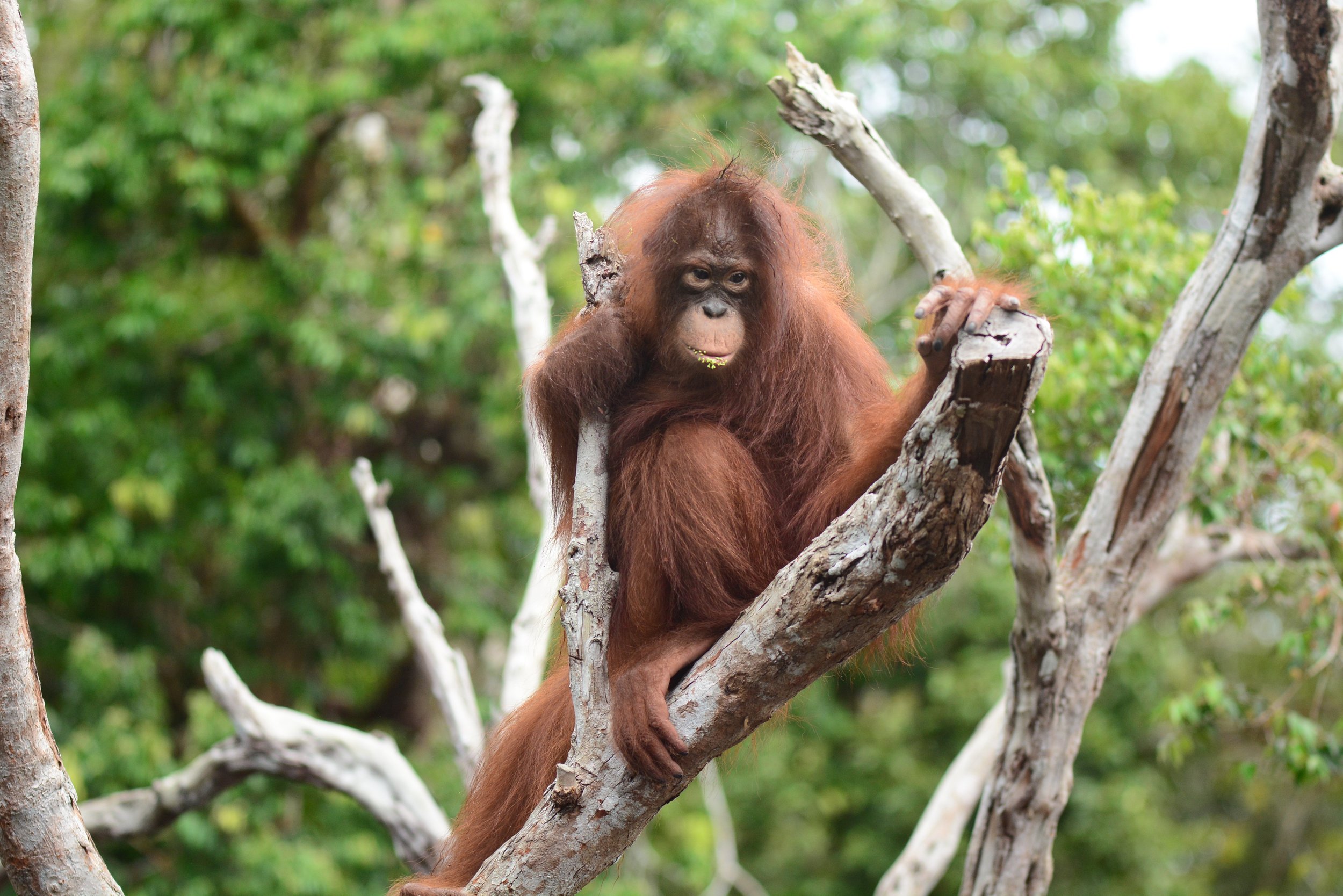The photograph depicts a majestic orangutan perched on a leafless, bare tree branch. His long, luxurious brown hair cascades down his body, almost creating an ethereal halo around him. His deep tan colored eyes, set above a round, black button nose, exude a sense of serious contemplation as he gazes downward, seemingly lost in thought. His left hand, displaying long fingers, grips tightly to the end of a sawn-off branch, while his right hand clasps another vertical branch, ensuring he maintains his balance. His curled feet are also secured around the middle of the branch. The background showcases a lush, towering forest with green leaves, though slightly blurred, adding a natural ambiance to the scene. The orangutan's serious and somewhat forlorn expression suggests a contemplative moment, perhaps as he studies the person taking the photograph. The overall scene is bathed in natural light, adding to the authenticity of the habitat, which may be a zoo enclosure with trees made to resemble natural branches.